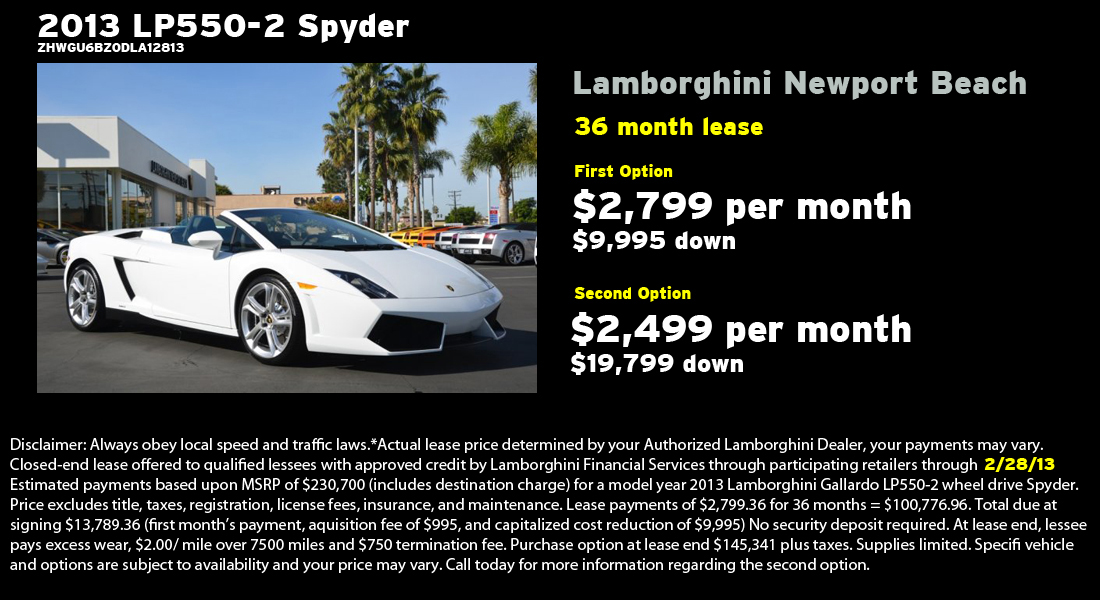The scanned advertisement features a sleek promotional graphic for a 2013 Lamborghini LP 550-2 Spyder. Displayed prominently on the left side is a striking photograph of a white convertible Lamborghini stationed against a backdrop that includes palm trees and a dealership, evoking a high-end ambiance. Above the car image, in white letters, the model and year "2013 LP 550-2 Spyder" are clearly highlighted. Below this, the advertisement details leasing options on the right: "Lamborghini Newport Beach" in gray text, followed by leasing terms in yellow - "36 month lease." The first option presented is "$2,799 per month with $9,995 down," and the second option is "$2,499 per month with $19,799 down." A long white paragraph of disclaimer information is situated at the bottom, detailing terms and conditions, prominently including the date "2/28/13" highlighted in yellow, consistent with the leasing terms' font. The ad's background maintains a slick black, underscoring the elegance and exclusivity associated with the Lamborghini brand.